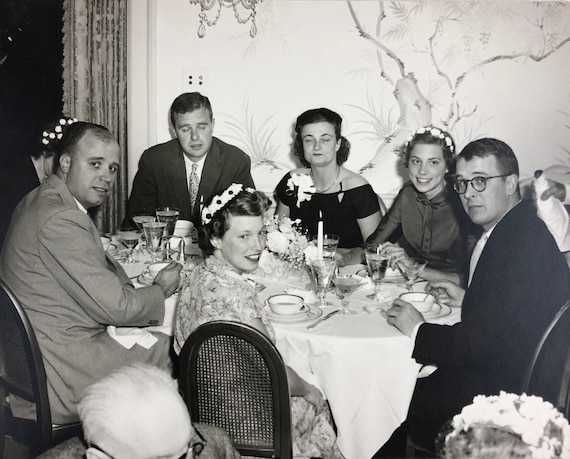This vintage black-and-white photograph, likely taken between the 1950s and early 1960s, captures a formal celebration, possibly a wedding or ballroom event. The scene centers around a round table draped in a white tablecloth, adorned with a floral centerpiece and lit candles. Seven people are seated, all in formal attire typical of the era: the men in suits with ties and the women in elegant dresses and hats. 

Starting from the bottom left of the image, an elderly gentleman with a bald head and gray hair, wearing black glasses, is partially visible. At the bottom right is a woman with blonde hair, wearing a white hat. 

At the table’s center, a woman sits facing the camera, smiling, with a white hat featuring black spots. To her left, a balding man in a gray suit glances sideways. Beside him, another woman’s hat with white spots is just visible. Moving right, a clean-shaven man in a darker suit sits with his eyes closed and mouth slightly open. Next to him, a woman with short hair and a black dress, possibly with a white corsage, also has her eyes shut. 

Further right, another woman smiles in a dark blue or black dress, with her arms partially exposed. She wears a hat trimmed with white flowers. To her right, a man in a black suit, wearing glasses and holding a spoon, appears unaware of the photo being taken. 

A waiter, holding a champagne bottle wrapped in a white napkin, is captured in motion on the right side of the image. In the background, the scene is set with ornate curtains, an elaborate chandelier with glass and ruby-like decorations, and a wall feature of a thin palm-like tree. The sophisticated ambiance is emphasized by the detailed decorations and the formal attire of the attendees.